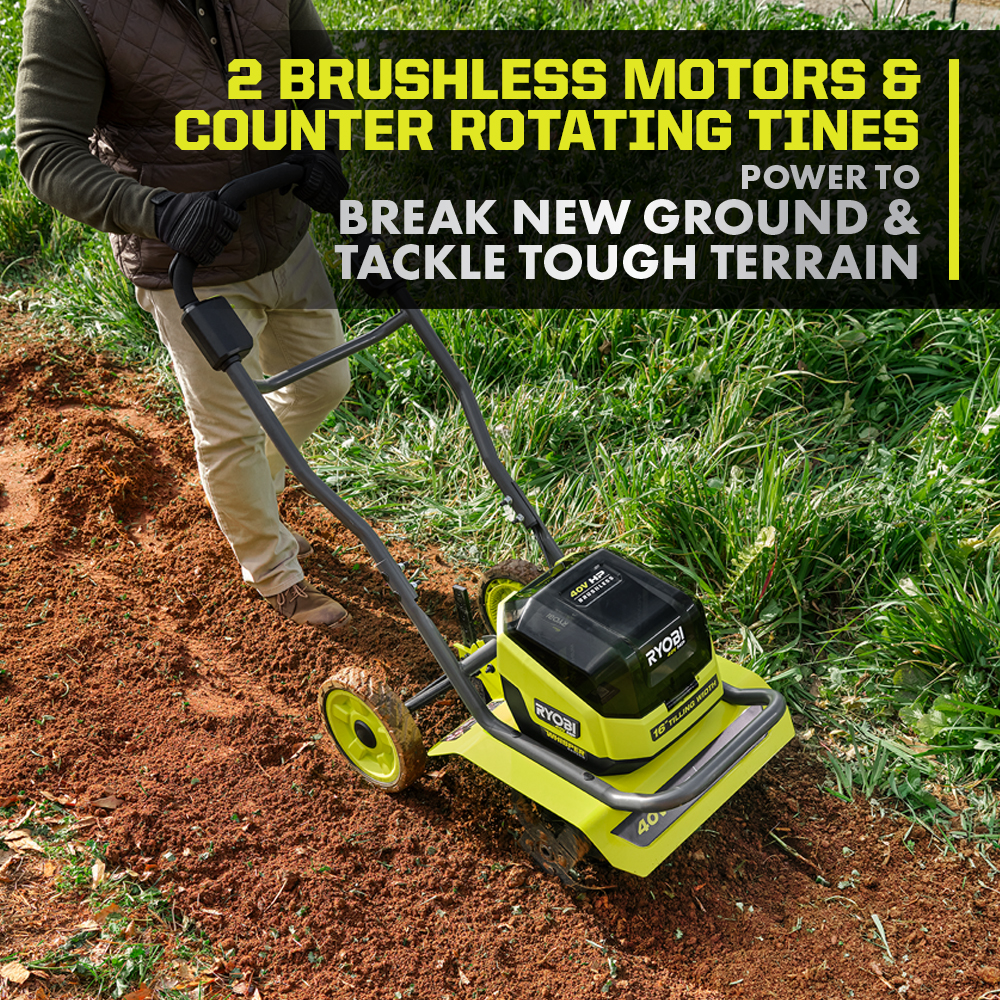The image is an advertisement showcasing a powerful garden tiller. The setting is outdoors, featuring a large dirt area in the foreground where the machine is actively being pushed through the soil, likely preparing it for planting crops, a garden, or flower beds. A man is operating the tiller, wearing khaki pants, brown work boots, a green and brown jacket, and black gloves. His attire suggests he is dressed for outdoor labor. In the background, there is an expansive area of long grass, contrasting with the tilled soil. Prominently displayed at the top of the image is a block of text in yellow, white, and gray: "Two brushless motors and counter-rotating tines. Power to break new ground and tackle tough terrain." The text highlights the tiller's features, emphasizing its capability to handle challenging terrains with ease.